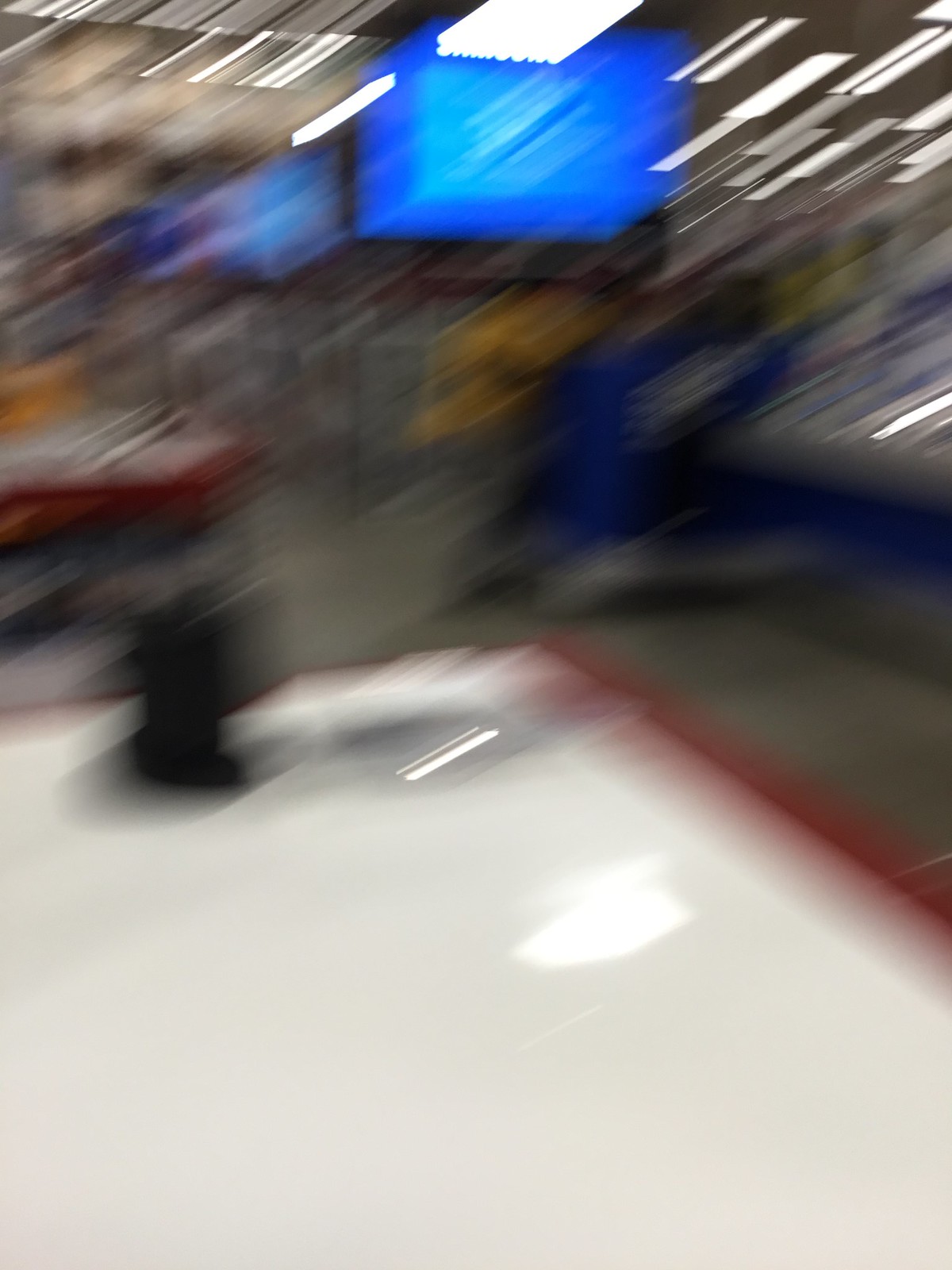The image depicts a game room featuring two air hockey tables, identifiable by their white tops and red borders. Adjacent to these tables, there is another game that involves throwing objects, indicated by angled targets visible in the background. The floor is gray, and the atmosphere includes various game-themed decor. Additionally, a black object sits near the corner of one of the air hockey tables, adding to the room’s detailed setting. Overhead, there is a telemonitor mounted on the ceiling, enhancing the immersive gaming experience.